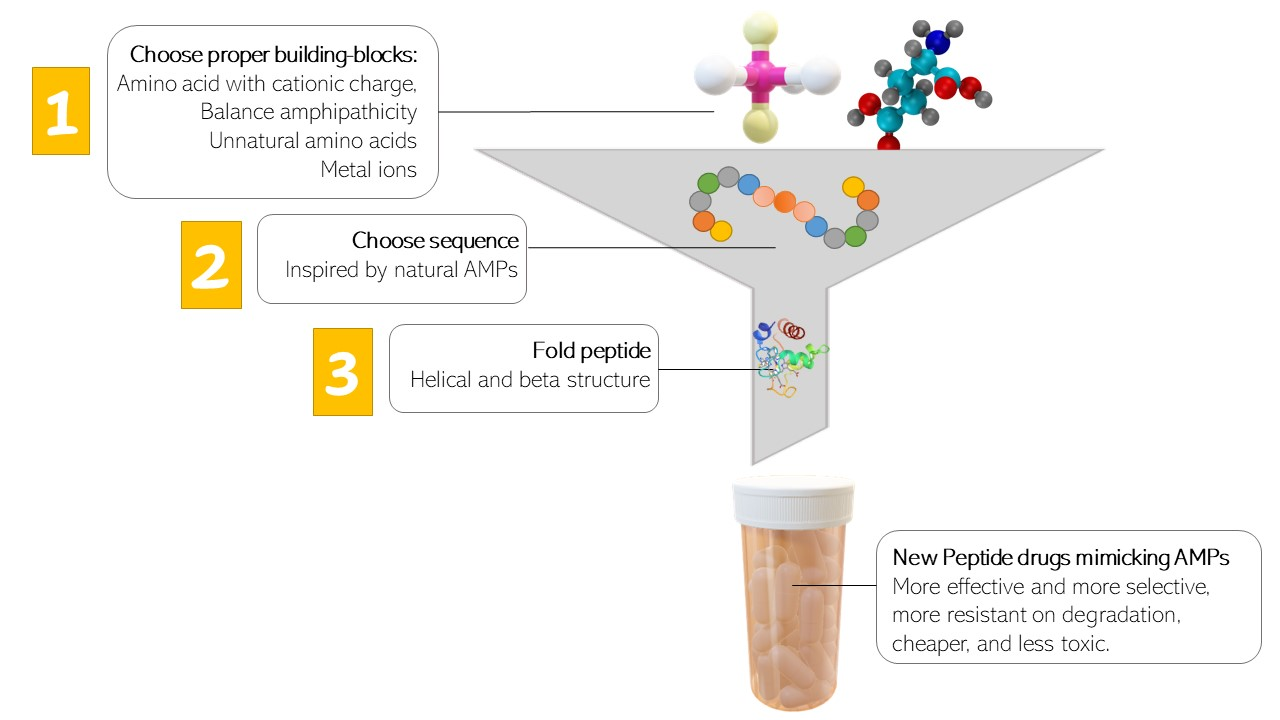The image depicts a detailed diagram, likely from a science or medical textbook, illustrating the process of creating new peptide drugs. At the center bottom, there is a pink pill bottle with a white cap, labeled to highlight the benefits of these new peptide drugs that mimic antimicrobial peptides (AMPs), including increased effectiveness and selectivity, resistance to degradation, reduced cost, and lowered toxicity.

Above the pill bottle is a funnel, representing the synthesis process. The funnel is visually split into three sections, each corresponding to a step in the peptide creation. In the first section, there are labeled building blocks—amino acids with cationic charge, amphipathicity, unnatural amino acids, and metal ions. The second section focuses on choosing sequences inspired by natural AMPs, depicted as a string of beads. The third section shows the folding process of the peptide into helical and beta structures.

Text boxes with yellow backgrounds and white numbers guide the steps, with additional explanatory text in white boxes with black lettering, providing a clear step-by-step breakdown of the synthetic process leading to the final product. The diagram not only educates on the creation of peptide drugs but also emphasizes their superior properties through visual and textual information.